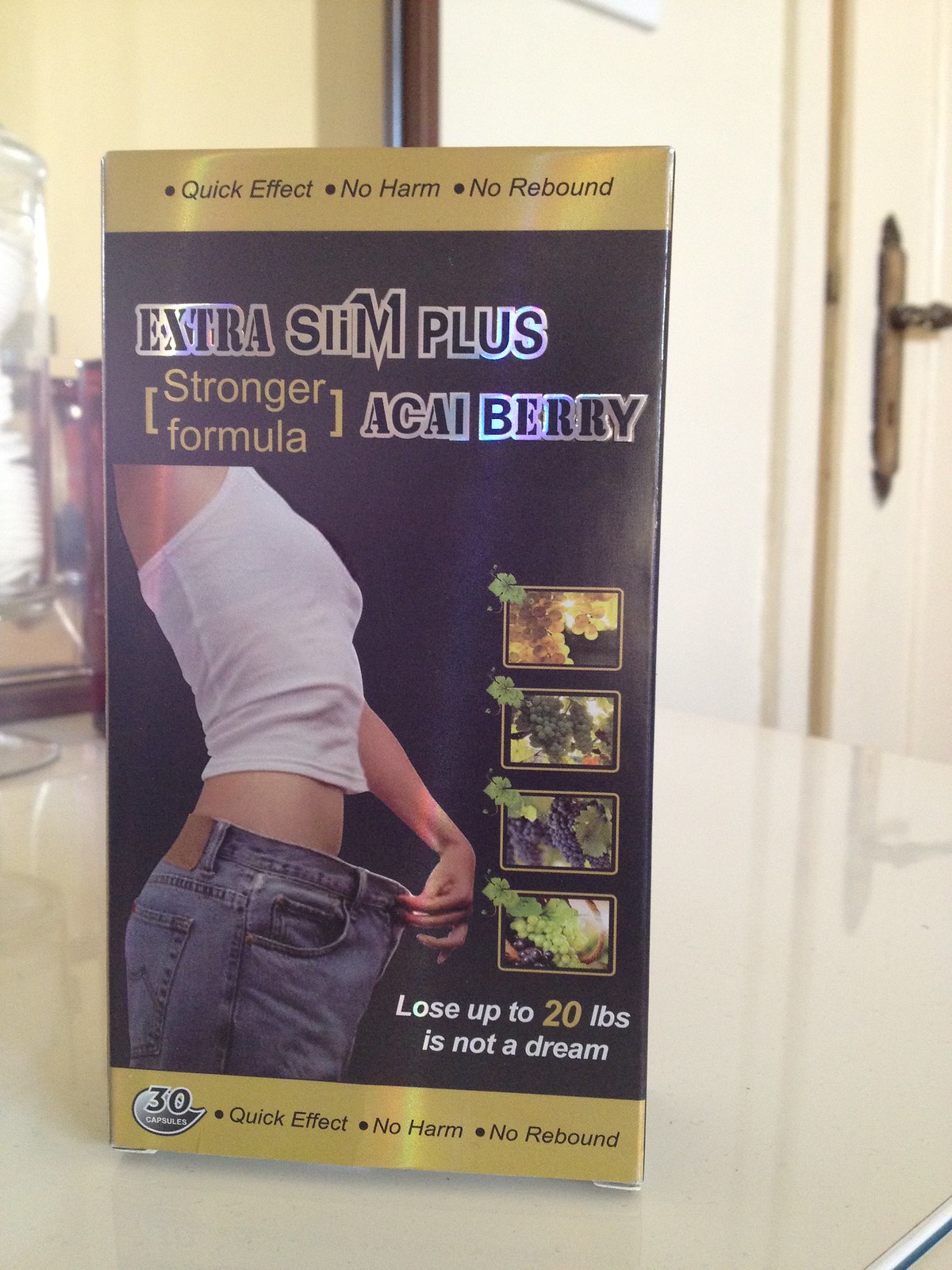The photograph features a product advertisement prominently presented against a striking black background. At the top, bold black text set against a gold band reads, "Quick effect, no harm, no rebound." The image is a dynamic blend of black, gold, and white fonts that capture attention.

Centrally highlighted in black font are the words "Extra Slim Plus," followed by "stronger formula" in gold font. Below this, "Ackie Berry" is displayed in black font.

Accompanying the textual elements is a vibrant image of a model dressed in a white cropped top and jeans, embodying the product’s promise of fitness and health.

The promotional text boldly states in white font "lose up to" followed by the number "20" in gold and then "pounds" in white, emphasizing that "It's not a dream." This assertion is reinforced by repeating the slogan "Quick effect, no harm, no rebound."

The product seems to be an exercise supplement, depicted in its packaging form. The image is set on a light-colored surface, with a subtle background hinting at a domestic setting, including a partial view of a white door with a bronzy handle.

This comprehensive layout not only presents the product’s features and benefits but also creates an appealing and aspirational visual narrative.